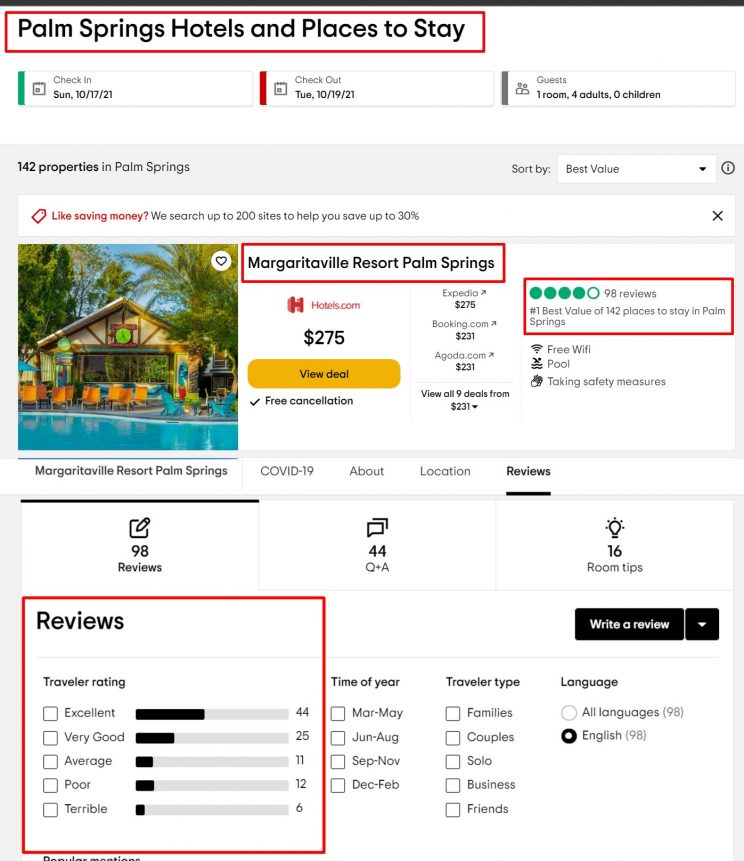The image is a screenshot from a travel website, featuring a header that reads "Palm Springs Hotels and Places to Stay." The overall design has a clean, white background with black text for easy readability. The focal point of the screenshot is a picture of the Margaritaville Resort, Palm Springs, positioned on the left-hand side, somewhat centered on the page. To the right of this picture, the resort’s name is prominently displayed along with its price, listed as $270, with a deal option of $75 each. 

The title "Margaritaville Resort, Palm Springs" is highlighted with a red rectangle. Adjacent to this, the resort's rating is also enclosed in a red square, showcasing a 4 out of 5-star rating. Beneath the rating, there are review summaries, again in red-bordered boxes, indicating the following: 44 excellent reviews, 25 very good reviews, and 6 terrible reviews.

Following these details, the site provides options for refining the search results, allowing users to filter choices based on various factors such as property type, time of year, traveler type, and language preferences.